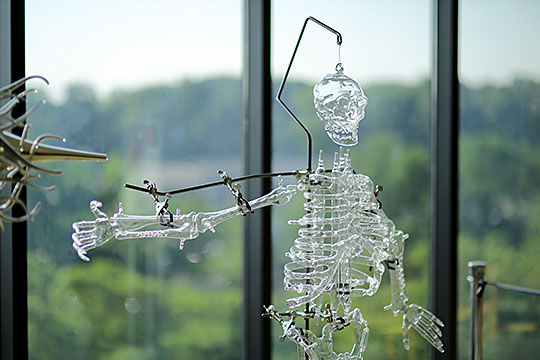The image depicts a meticulously crafted skeleton made of clear glass or plastic, showcased inside a building. The skeleton is supported on a sturdy metal stand and is further stabilized by a wire frame with multiple clamps, ensuring its upright position and the extension of its right arm. The head of the skeleton is subtly suspended from a clear plastic string. The display is prominently set in front of large windows with metal dividers, offering a serene view of a green, forested area under a blue sky with scattered clouds. In the background, beyond the skeleton, there is a stanchion with a velvet rope, suggesting that this is part of a modern art exhibit, possibly in a gallery. To the left of the skeleton, a glimpse of stainless steel adds to the contemporary setting. The overall scene captures a blend of intricate art and a natural backdrop, emphasizing the juxtaposition of man-made and natural beauty.